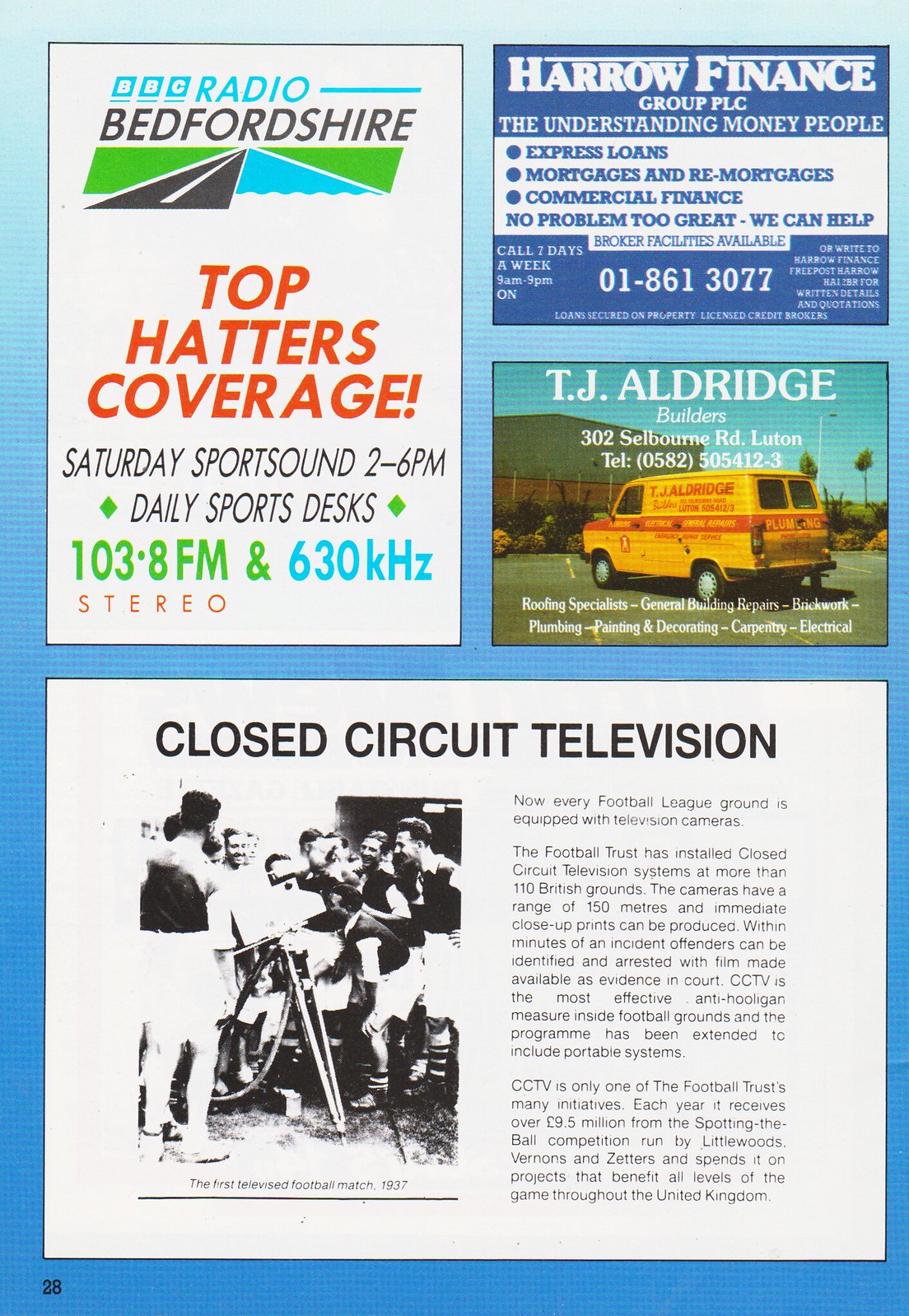This image depicts page 28 from a magazine, filled with four distinct advertisements against a powder blue gradient background that fades from darker to lighter at the top. The first ad in the top left corner promotes Radio Bedfordshire, featuring a logo with a drawn road and green grass. It details "Top Hatters Coverage" for Saturday sports from 2 to 6 p.m., airing on 103.8 FM and 630 kHz stereo. In the upper right corner, there is an ad for the Harrow Finance Group PLC, tagged as "The Understanding Money People," offering various financial services including loans and mortgages. Below it, a third ad for TJ Aldridge features an image of a yellow van with a red stripe, pertinent to a plumbing company. The bottom of the page presents another ad headlined "Closed Circuit Television," showcasing a historic scene from the first televised football match in 1937, with text positioned to the right of the photo, which depicts soccer players surrounding a TV screen.